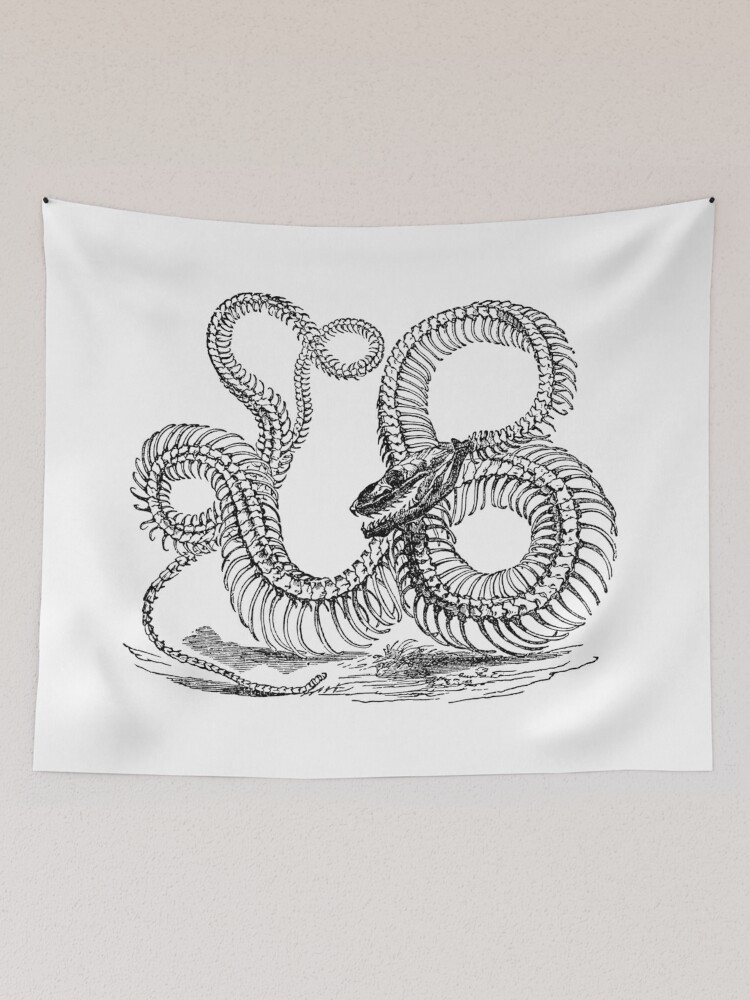The image depicts a detailed black and white ink drawing on a cloth-like canvas, which is pinned to a grayish-tan wall by two small pins. The drawing showcases the skeletal remains of a very large snake, possibly resembling an anaconda, though no wings are present to suggest it might be a dragon. The skeleton loops and twists intricately, forming various curves and bends, and even makes an eight-like shape around the head area, which is positioned toward the left side of the canvas. The snake's head, prominently black with visible rows of teeth in the jaws, contrasts against the white background. The majority of the snake's skeleton is thick, but it tapers down to a very tiny tail resembling the size of a pencil. Ground elements like grass and shadows are illustrated at the bottom of the canvas, adding depth to the scene. Dust appears to rise from the skeleton, enhancing the dynamic and lifelike quality of the artwork.